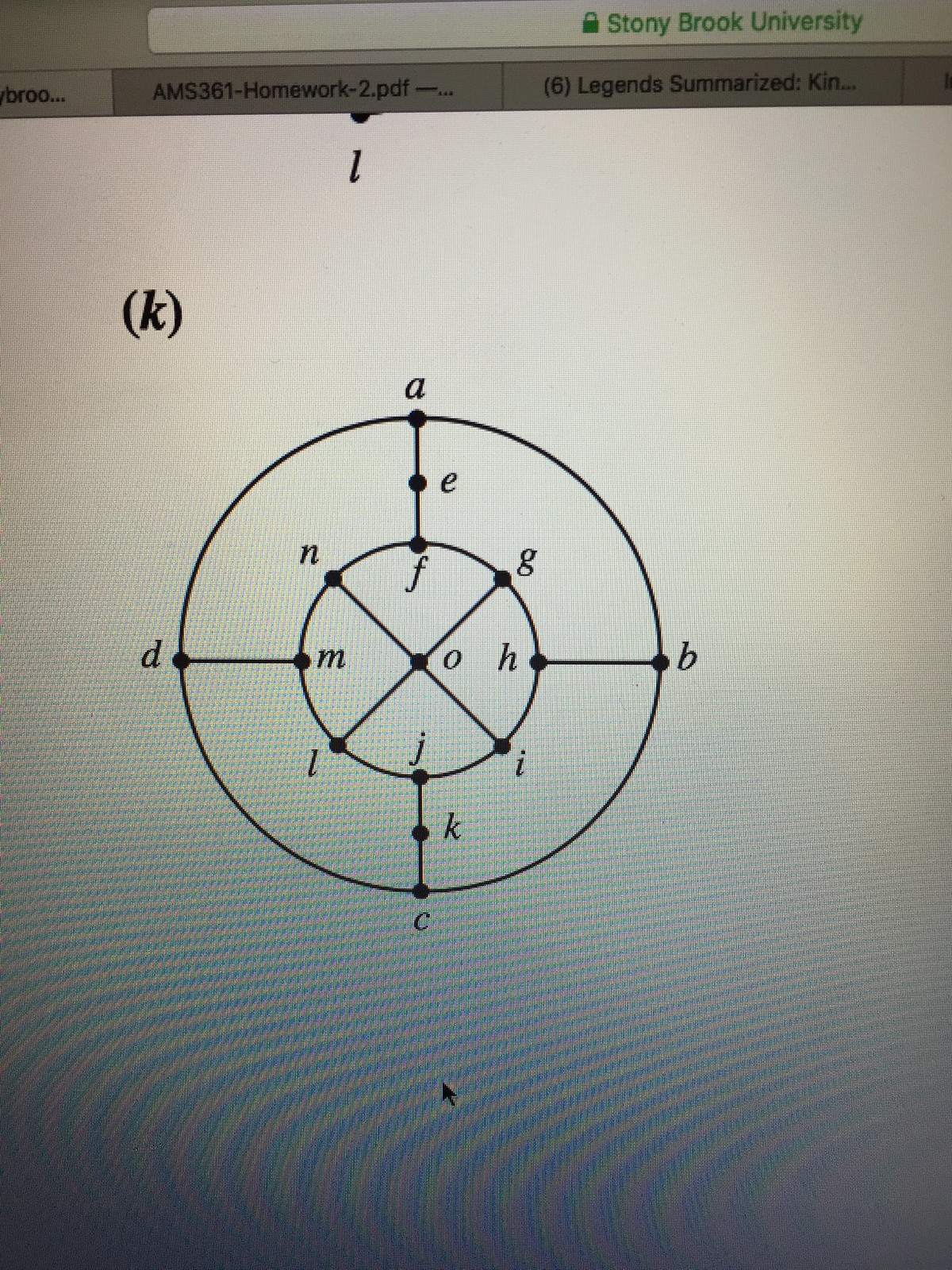Photograph of an illustration: At the top of the photograph, the words "Stony Brook University" are prominently displayed. The illustration appears on a mostly white background, possibly paper. Below the main portion, there is a blue-colored section that displays visible pixels, suggesting the image might have been captured from a computer monitor. A black pointer is evident towards the lower part of the screen.

The illustration itself consists of two concentric circles with an 'X' shape intersecting them. Surrounding the outer circle are the letters A, B, C, and D. Within the inner circle are the letters N, G, I, and L. On the lines of the 'X' within this inner circle, the letters M, H, O, and J are arranged, and there is a 'K' in parentheses at the top of the 'X'.